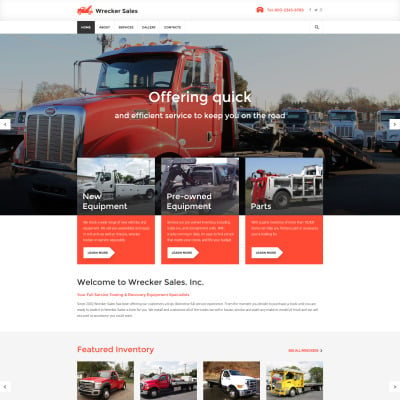A webpage displaying record sales is shown in the upper left corner, alongside a telephone number in red on the top right, which is slightly blurred. Below that, a horizontal menu bar spans across, although some menu items are not legible. However, 'Home' and 'Dealer' are among the visible options. To the right of the menu bar, there's a search bar and button.

Dominating the webpage is a prominent image of a red diesel tow truck with a flatbed. Centered on the image, white text reads, "Offering quick and efficient services to keep you on the road." The scene appears to be winter, with bare trees and a blue sky suggesting early morning or evening light. In the background, to the right, several identical white pickup trucks are visible, positioned behind the red tow truck.